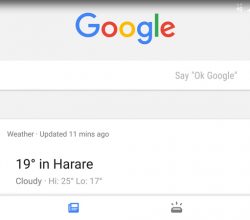Screenshot of a Google Search Interface: The image captures a screenshot from the Google search page. At the top, the Google logo is prominently displayed with its customary color scheme: a blue "G," a red "O," a yellow second "O," a blue second "G," a green "L," and a red "E." Directly beneath the logo is the prompt, "Say 'OK Google,'" indicating the voice search functionality.

The weather update, last refreshed 11 minutes ago, reports the current conditions in Harare, the capital of Zimbabwe, spelled out as H-A-R-A-R-E. The weather details show a temperature of 19 degrees Celsius, with a cloudy sky. The forecasted high is 25 degrees Celsius, and the low is 17 degrees Celsius.

The image strictly consists of text and graphic elements; there are no photographic components present. It is devoid of any living beings such as people, animals, or birds. Additionally, there are no natural elements like plants, flowers, or trees, nor any man-made structures such as buildings, bridges, or bodies of water. The image also lacks any form of transportation including cars, boats, motorcycles, bicycles, helicopters, or airplanes.